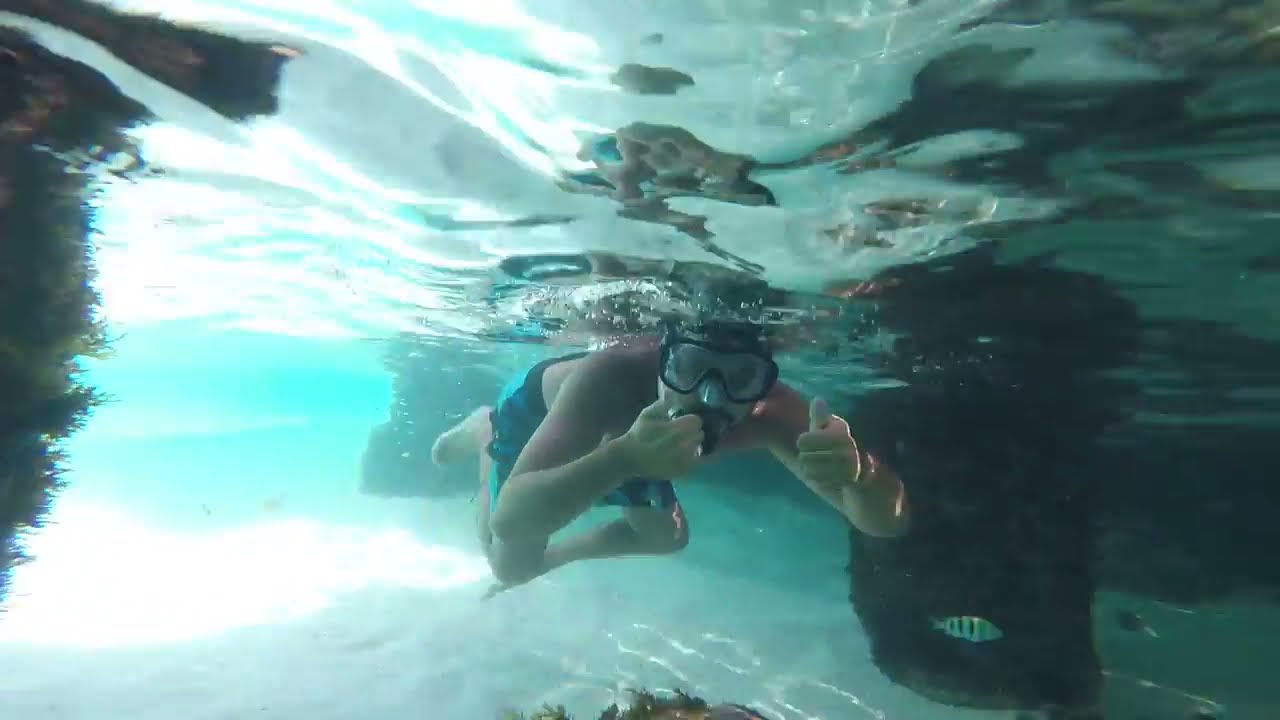This underwater photograph captures a light-skinned man snorkeling in crystal-clear, shallow waters. Central to the image, he dons blue swim trunks and black-framed goggles, with a snorkel protruding from his mouth. He appears to be swimming towards the foreground, his gaze directed ahead. The water above him is highly reflective, displaying ripples that hint at the surface just above his head. Surrounding the snorkeler, the underwater landscape features white sand, scattered rocks, and vibrant coral formations, primarily to the left and right sides of the frame. These coral structures, resembling large cylindrical pillars, are adorned with algae and various forms of sea life, creating a vibrant, immersive scene reminiscent of an aquarium. In the background, light pierces through the water, casting a brighter glow to the left side of the photograph.